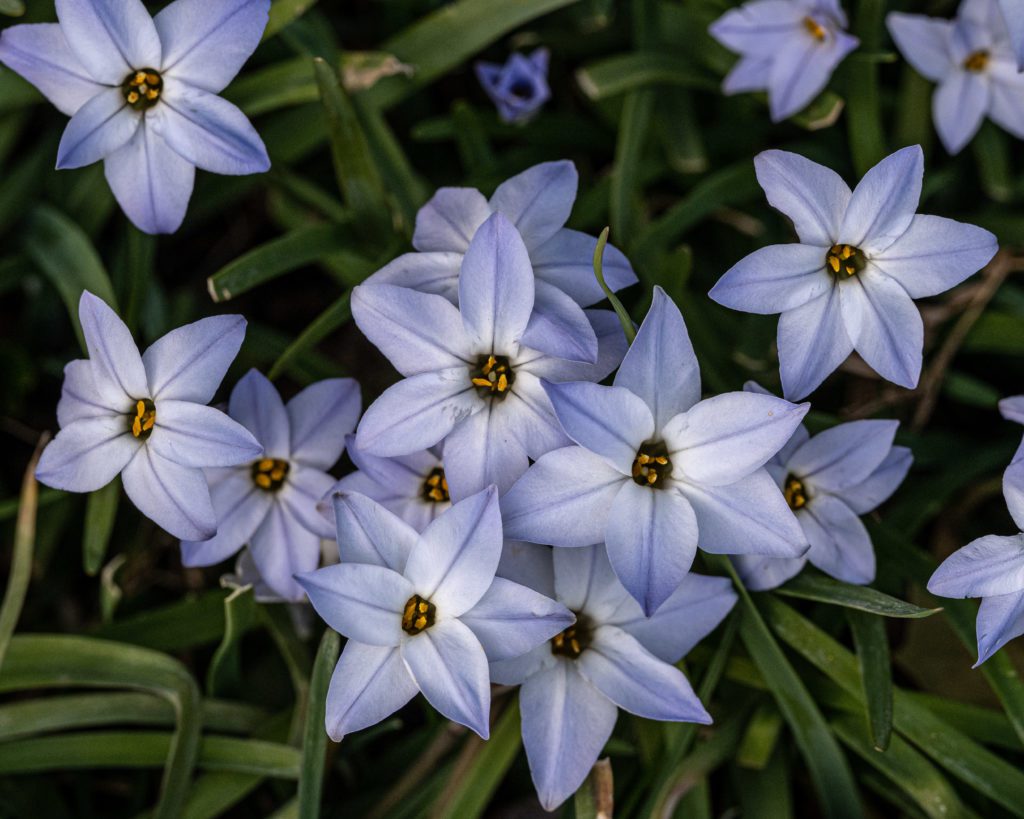This is an overhead view of approximately 14 to 15 white flowers, each featuring six oval-shaped petals with a crease down the center, creating a realistic yet painterly effect that could easily be mistaken for a photograph. The petals are white with a subtle greyish bend in the middle. The flowers are primarily clustered in the bottom center of the image, but some can be found in the upper left and right corners as well. Each flower has a dark brown center adorned with three irregular yellow dots, arranged in a way that almost gives a resemblance to a human face. The flowers are set against a tangled backdrop of long, thin, ribbon-like green leaves that crisscross in all directions, beneath which the background fades into a deep black, adding to the intrigue of the composition.